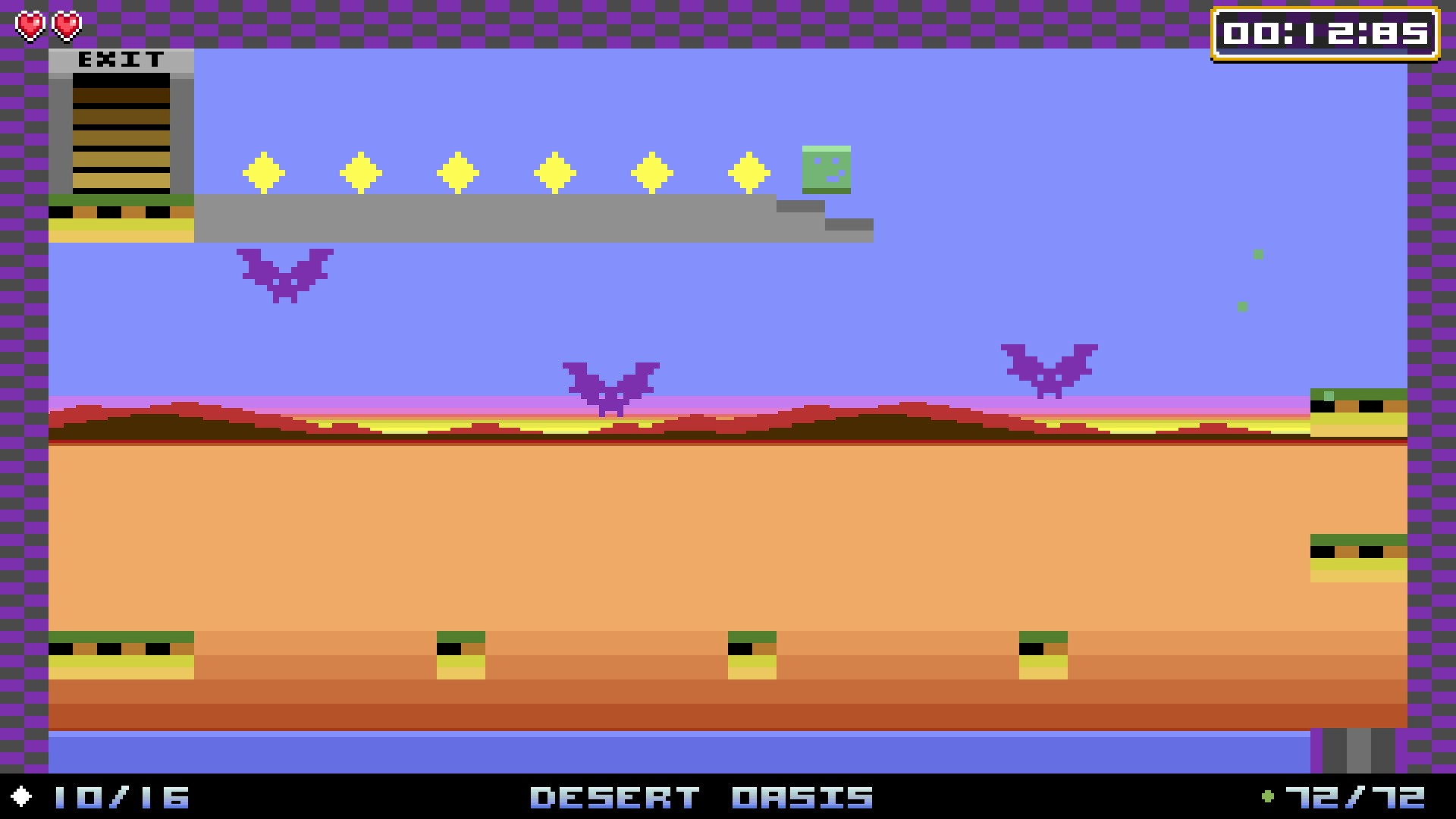This is a horizontally rectangular, color photograph resembling a retro video game screenshot. The image is highly pixelated and vibrant with colors. A border comprised of alternating lighter and darker purple rectangles decorates the top and left-hand sides, culminating in a solid black border at the bottom with white text. The bottom border prominently displays "10/16 Desert Oasis 72/72." Within the top-left corner, two red hearts can be seen on the border, alongside an "Exit" sign with green and brown hues. In the top-right corner, a timer reads "00:12:85" in white text on a black background.

The scene depicts a desert landscape with vivid, reddish-pink mountains in the background against a blue sky transitioning to yellow at the horizon. Sand stretches out in the foreground, infused with pixelated details. Three purple bats, characterized by their wing-flapping motion, are flying in the sky. Additionally, a grey bar adorned with yellow diamonds and a small green square appears over the sky, enhancing the retro, pixelated aesthetic of the scene.